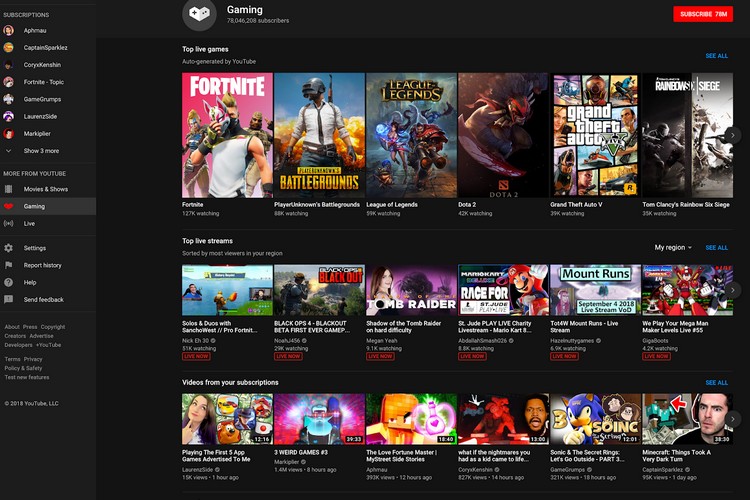The screen displays a "Gaming" section header with a distinctive logo on the left comprising two squares—one containing a plus sign and the other with two dots. To the right of the logo, the text "Subscribe 78m" is prominently displayed in white on a bright orange background.

On the left-hand side of the screen, a vertical list of categories extends from top to bottom, starting with "Subscriptions" at the top and ending with "More from YouTube" at the bottom. The screen is currently focused on the "Gaming" category, situated between "Movies & Shows" and "Live."

The primary content area on the right-hand side, set against a black background, features three rows of games, each with six games for a total of 18. 

- The top row is labeled "Top live games auto-generated by YouTube," with a blue "See All" link on the right.
- The middle row shows "Top live streams sorted by most viewers in your region," with a region filter indicated in white and another blue "See All" link on the right.
- The bottom row is titled "Videos from your subscriptions," also accompanied by a blue "See All" link above the top-right video.

Below each category title and preceding the list of games, there is a segment of small, light gray text.